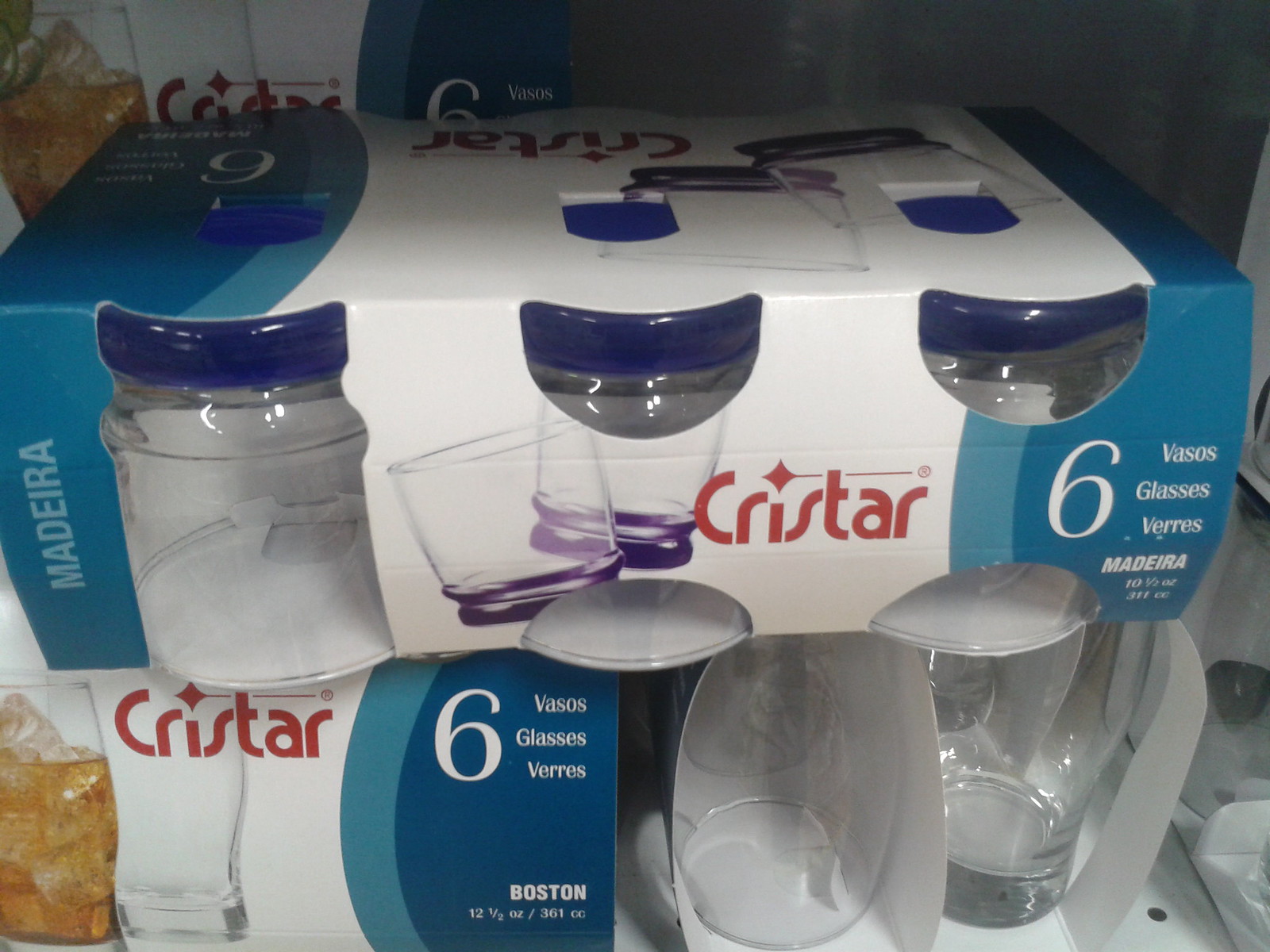A close-up image of newly purchased Cristar glassware in a store shelf, showing packages of clear drinking glasses. The shelf displays multiple multi-packs, primarily showcasing small, round, clear glasses and glasses with blue-colored bottoms. Each multi-pack contains six glasses. The cardboard packaging is light blue on the ends with a white stripe in the center, featuring the Cristar brand name in red letters. The packages are stacked, one on top of the other, and have labels indicating that each glass is 12.5 ounces in size. The photo is taken in what appears to be a white countertop kitchen setting. "Boston" and "six vassals" are also written on the packaging.